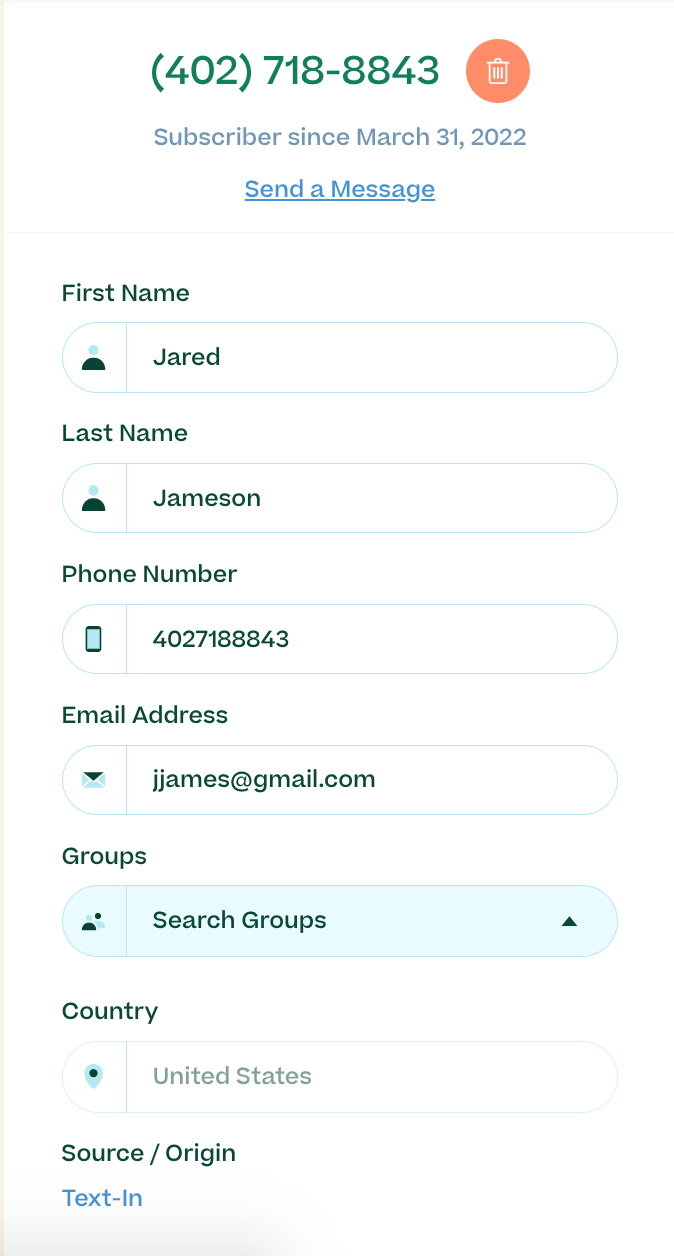This digital image displays a user profile interface. At the top, prominently featured, is a phone number: 402-718-8843. Adjacent to it, there is a trash button icon, represented by an image of a trash can within an orange circle. Below this, there is a subscription status noting "Subscribers since March 31st, 2022."

Further down, a blue "Send a Message" button is visible. Underneath this, user details are listed, including the first name "Jared" and last name "Jameson," alongside the repeated phone number 402-718-8843. An email address, jjames@gmail.com, is prominently displayed as well.

The user interface also includes a "Groups" tab accompanied by a "Search Groups" button. Beneath this, there is a section for "Country," with "United States" being selected. Following that, there is a section labeled "Source/Origin," with the final noteworthy text being "Text In."